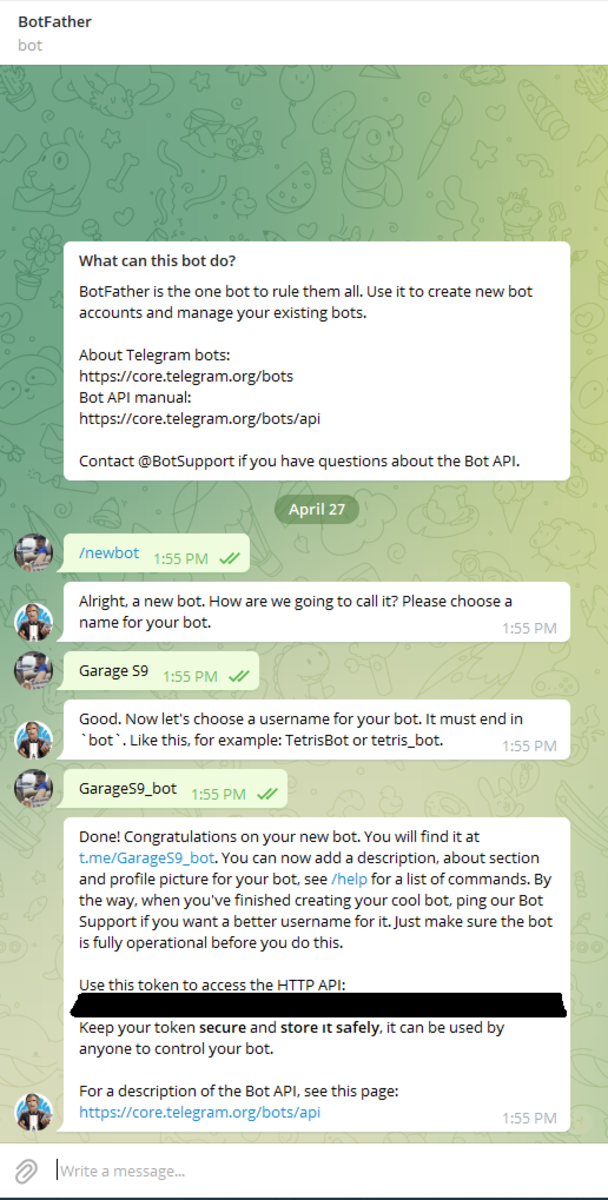This screenshot captures a detailed view of a Telegram conversation interface. The image features a white border about an inch thick surrounding the chat area. Along the top is a slim black line. In the top left corner, "BOT FATHER" is displayed in bold, with "BOT" written below it in smaller text. 

The background transitions from dark green on the left side to progressively lighter shades of green as it moves to the right, eventually turning white towards the bottom. The dark green background is decorated with playful drawings of dogs, pizza slices, and various small icons.

Approximately two inches from the top, there is a white rectangle containing black text. The text reads:
- "What can this BOT do?"
- "BOT FATHER is one BOT to rule them all. Use it to create new BOT accounts and manage your existing BOTS."
- "About Telegram’s BOT features."
- "Contact BOT support if you have questions."

In the center of the darker green area, a tab with white text reads "April 27."

On the left side of the page are profile icons or thumbnails, each corresponding to different users. To the right of these icons, message tabs indicate ongoing conversations. For one user, the message "new BOT" is shown at 1:55 PM, accompanied by two green check marks indicating the message has been read. The screenshot documents six exchanges: five brief one-line messages, and one final, much longer conversation spanning two paragraphs.